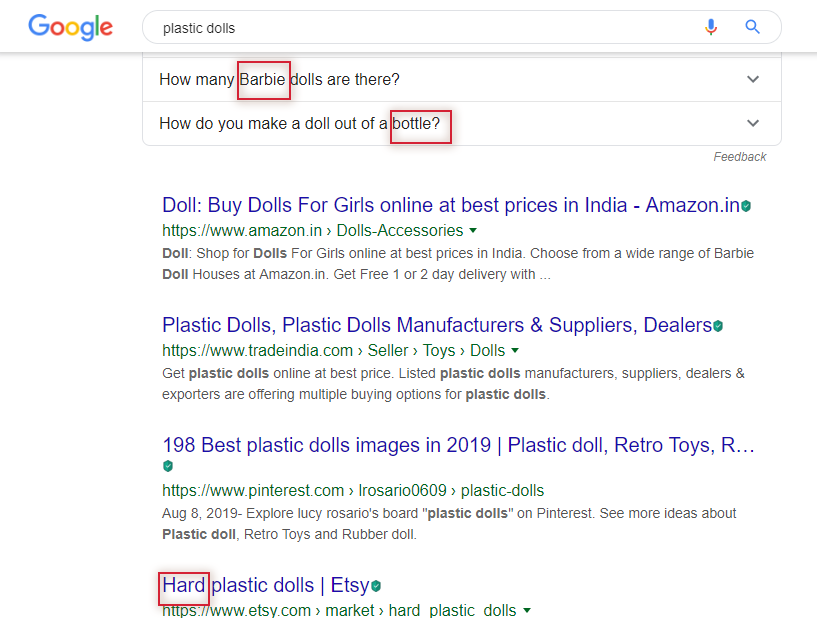In the image, a Google search page is displayed on a computer screen. At the top of the page, within the search bar, the text "plastic dowels" is visible, located adjacent to the multicolored Google logo. Below the search bar, the first suggestion reads "how many Barbie dowels are there," with the word "Barbie" highlighted by a red rectangle. The second suggestion states, "how do you make a dowel out of a bottle?" with "bottle?" enclosed in a red rectangle.

Following these suggestions, four search results are listed. Each result features a blue clickable title, accompanied by a green clickable URL below it. The first result reads, "Buy dowels for girls online at best prices in India," linked to Amazon.in. The second result is titled, "Plastic dowels, plastic dowels manufacturers and suppliers, dealers." The third result, positioned at the bottom, mentions "198 best plastic dowel images in 2019." The fourth and final result is from Etsy, labeled "hard plastic dowels," with the word "hard" also surrounded by a red rectangle.